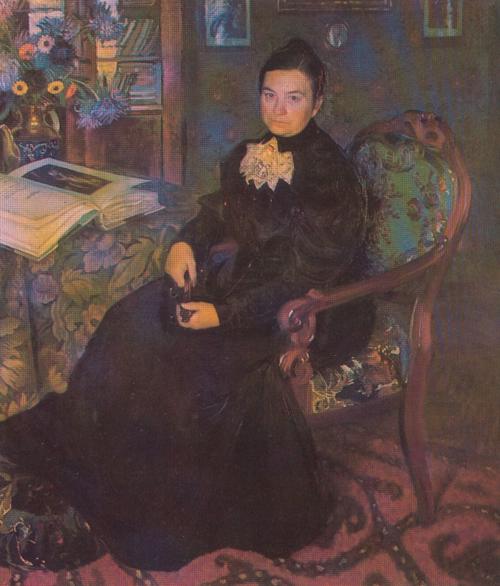The artwork appears to be an old, possibly Renaissance-era painting given a modern holographic or rainbow filter. It depicts a middle-aged or older woman with fair skin and dark hair pulled back into a tight bun. She is seated in an elaborately embroidered wooden chair, facing left but gazing directly at the viewer. She wears a long-sleeved, high-necked black dress adorned with intricate gold detailing and a white lace ruffle at the collar.

The woman is positioned next to a table draped with a floral-patterned cloth. On the table lies an open book with visible text on the left page and a colorful illustration on the right. Beside the book stands a beautifully decorated vase filled with a vibrant array of flowers, including sunflowers, and other yellow, orange, white, blue, purple, and pink blooms.

The background features a green wall adorned with small pictures and portraits, while a bookshelf can be seen behind her. The floor is covered with a prominently red carpet featuring intricate black lines and swirling patterns. The overall composition and rich details evoke a blend of classic and contemporary artistic elements.